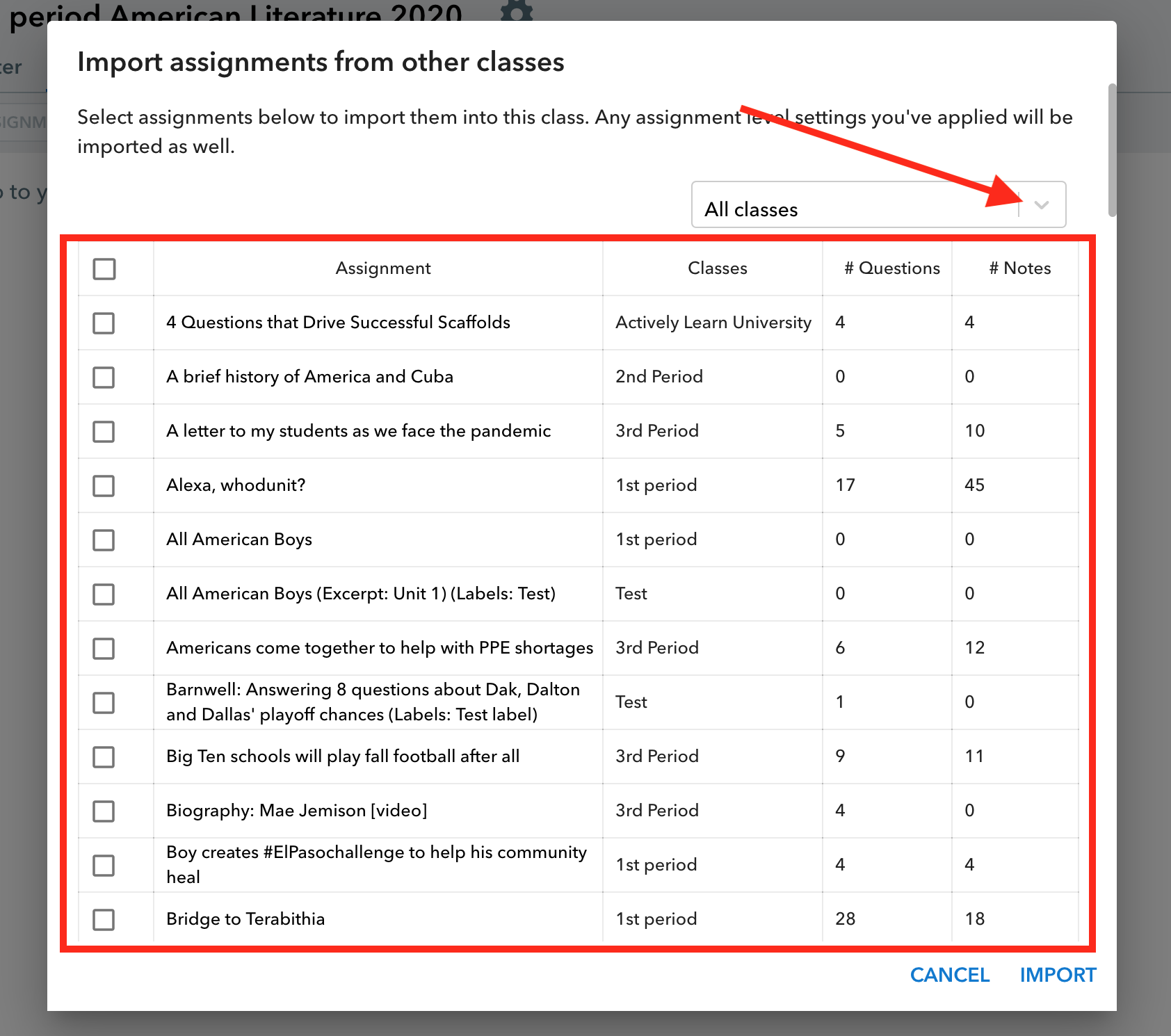The image showcases an online educational platform interface. The background features a gray square with the text "Period American Literature 2020" prominently displayed at the top. Dominating the screen is a large white box with instructions: "Import assignments from other classes. Select assignments below to import them into this class. Any assignments, level settings you've applied will be imported as well." 

In the top right corner, there's a narrow box labeled "All classes" accompanied by a drop-down arrow, highlighted by a long red arrow originating from the top and pointing towards this drop-down menu. Below this, there's a list labeled with "Assignments," "Classes," "Questions," and "Notes," encased within an orange border for emphasis.

To the left of this list, there are small, empty squares aligned beside each category, indicating selection options. A series of entries follow, specifying various assignments and class periods, including: 12 assignments, Activity Learning, Activity Learn University, second period, third period, first period (repeated multiple times), test, third period, and so on. The layout is styled in a structured, organized manner, supporting easy navigation and selection for the user.